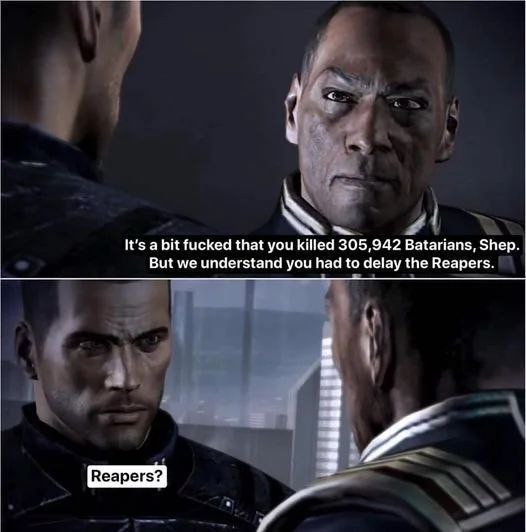The image consists of two horizontally stacked screenshots, likely from a video game or a movie clip. The top screenshot features two dark-skinned men with serious expressions. The man on the left has his back slightly turned, revealing just the right side of his face, neck, and shoulder, dressed in black. The man on the right is more fully visible, donning a jacket with white stripes along the collar. This upper image has white text over a black background in the bottom right corner that reads, "It's a bit fucked that you killed 305,942 Batarians, Shep, but we understand you had to delay the Reapers."

The bottom screenshot reverses the perspective, showing the front of the man on the left, who now reveals a serious expression and very short brown hair, clad in a black collared jacket. The man on the right is now seen from behind. In this image, there’s a small white rectangle with black text positioned on the neck of the man on the left, which says, "Reapers?"